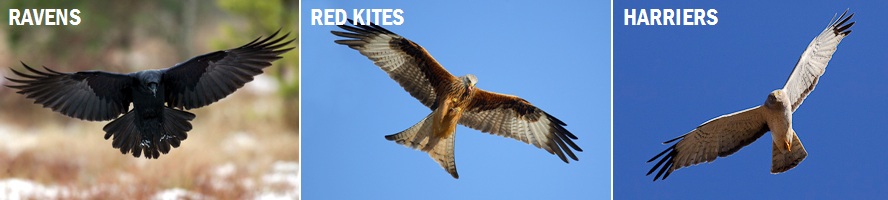This is a detailed photo collage, akin to something you might find in a National Geographic magazine or a documentary. The collage is rectangular and divided into three sections, each showcasing a different bird in flight against varied backgrounds, with text labels in large white font in the top left corners.

On the left, it says "Ravens." The image features a large black bird with fully outstretched wings and tail feathers, captured in mid-flight over a blurry, forest-like background with shades of brown and green suggesting trees and plants.

In the middle, it says "Red Kites." This section has a light blue sky backdrop, depicting a bird with a light brown body, triangular light and dark gray tail feathers, and wings that are dark near the body, transitioning to white, and ending with darker tips. The bird appears to be flying high, with its wings spread wide.

On the right, it says "Harriers." Against a darker blue sky, this part shows a predominantly white bird in flight. The harrier’s wings are fully extended, featuring black tips, and its tail feathers exhibit a darker color.

The collage is a striking capture of these birds in their natural flight, emphasizing their distinctive features and the different sky backgrounds.